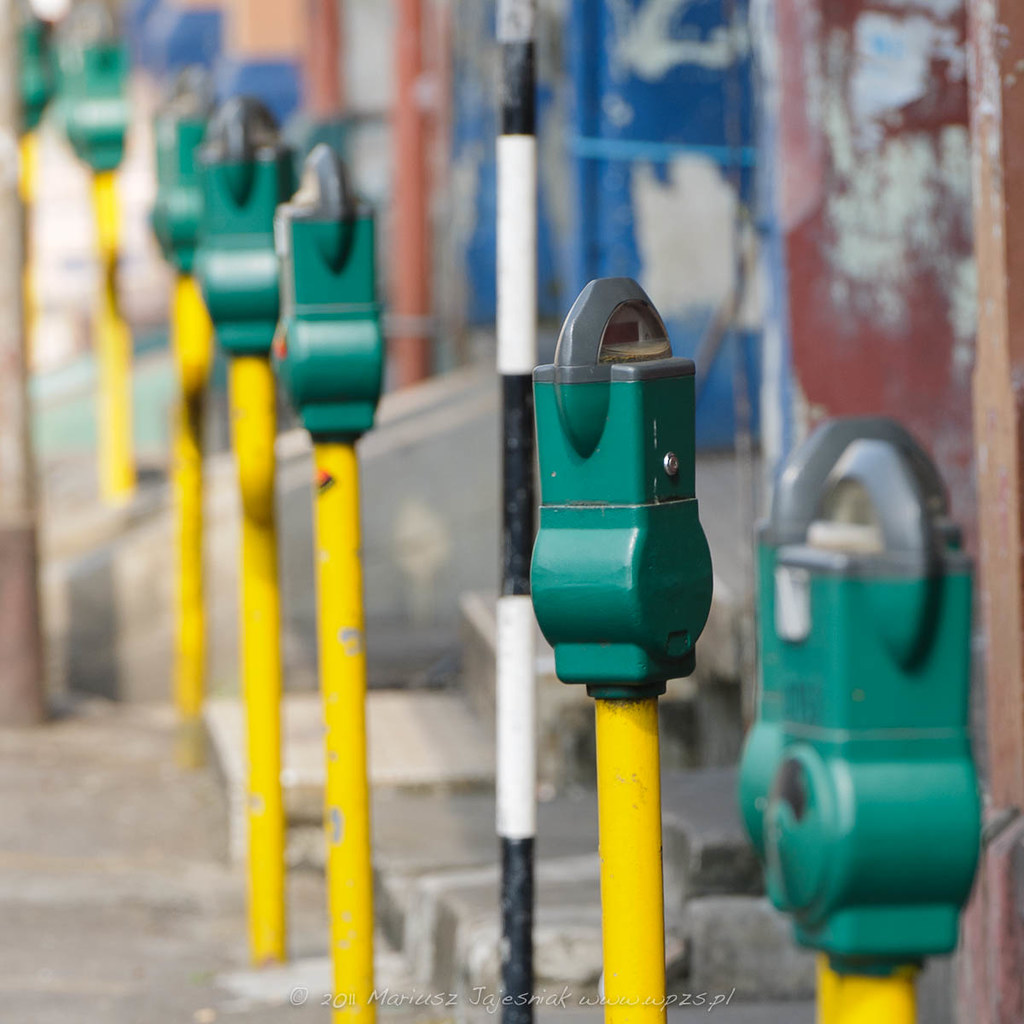The image captures a long row of parking meters along a sidewalk. These meters are characterized by bright yellow poles connecting them to the ground and hunter-green housings with small gray arches at the top, showing signs of wear with chipping yellow paint revealing gray underneath. There are a total of seven meters visible in the image. Past the first two meters, a taller black and white pole with a striped pattern extends from the ground. In the background, a rusted metal wall and several weathered, peeling walls with patches of red, blue, and orange paint hint at a run-down area in need of maintenance. The image has an outdoor setting and showcases an urban environment with the meters standing out against the faded, dilapidated backdrop.